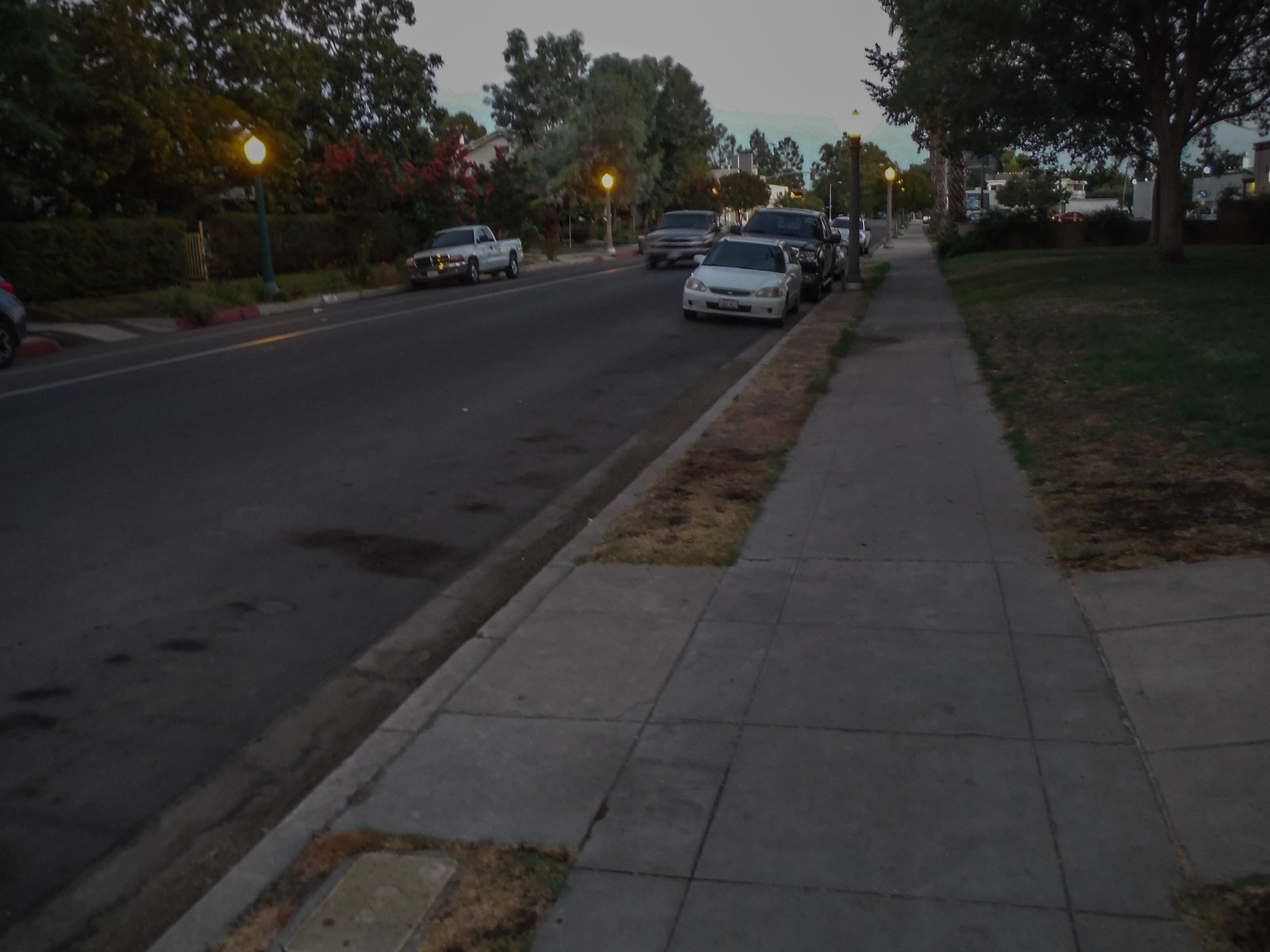The image captures a nighttime street scene from the perspective of someone standing on a sidewalk. The atmosphere is dim, with muted colors that emphasize the darkness. The camera is pointed down the length of the sidewalk, which extends straight into the horizon. 

To the right side of the image, a driveway begins, leading up to what is likely a house, while the driveway merges into the road on the left-hand side of the photo. The street is lit by three street lights; two are situated on the east side of the road, and the other two on the west side.

Parked along the curb on the east side of the street are a white car followed by a black pickup truck. Across the street, on the west side, another white pickup truck is parked. In the middle of the road, blurred by motion, a dark-colored SUV or pickup truck approaches the camera.

The yards of the houses lining the east side of the sidewalk are patchy, featuring grass interspersed with dark dirt spots. Notably, the yard directly to the east hosts a large oak tree. The horizon and the west side of the street are dotted with numerous trees. A house on the west side is obscured by a tall hedge, approximately six feet high. Near the road, lining the sidewalk, there are plants and trees that appear to be crape myrtles with red buds.